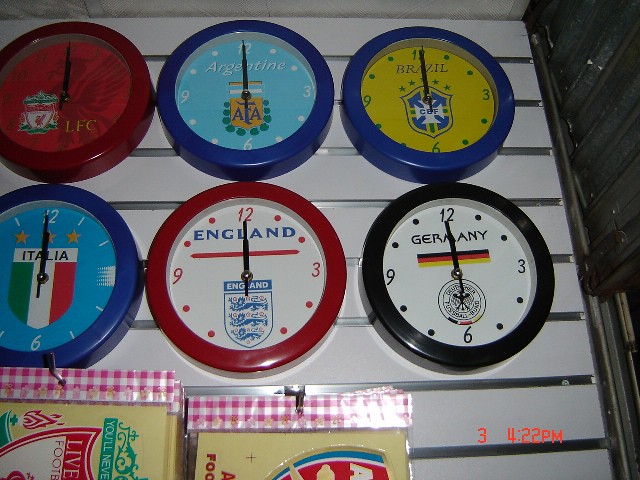The angled color photograph captures a store display featuring six themed wall clocks mounted on a white slatted wall with silver grooves, designed for hanging merchandise hooks. Each clock vividly represents a different soccer team with accompanying national crests: LFC, Argentina, Brazil, Italia, England, and Germany. The clocks are arranged in two neat rows of three, each clock face distinctly colored and marked at 12, 3, 6, and 9 with dots in between, and all hands pointing to 12 o'clock. The top row features a red clock, a light blue clock with 'Argentina,' and a blue clock with a yellow face labeled 'Brazil.' The bottom row displays a light blue clock with 'Italia,' a red-framed clock labeled 'England,' and a black, Germany-themed clock. Below the clocks, a peek of red-and-white checkered packaging is visible, suggesting additional soccer-related merchandise. In the bottom right corner, there's a timestamp reading '3 4 22 p.m.' in a digital font, indicating the photo's date.